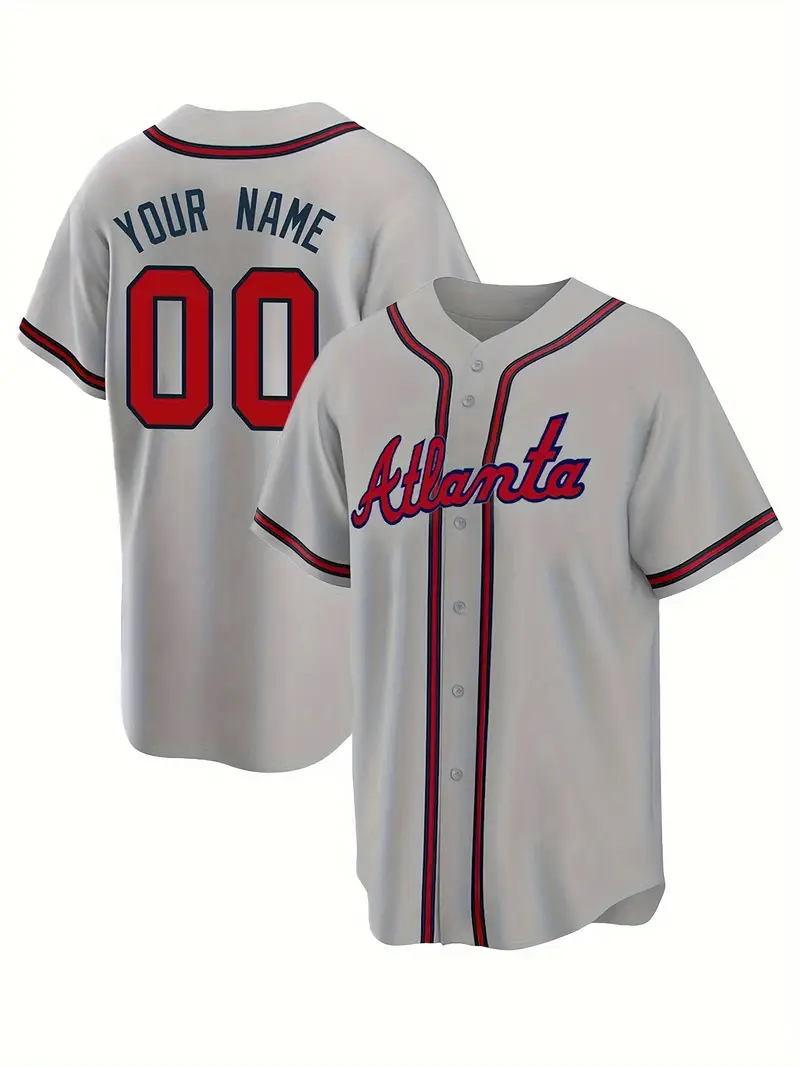This image showcases an official Atlanta Braves baseball jersey. The jersey features a soft gray hue and a front adorned with the word "Atlanta" written in elegant, red cursive italics. The front of the jersey is accentuated with bold red piping that vertically runs alongside the button placket. Notably, the back of the jersey includes space for customization, allowing fans to personalize it with their own last name. The overall design marries both classic and contemporary elements, making it a stylish and meaningful piece for any Braves enthusiast.